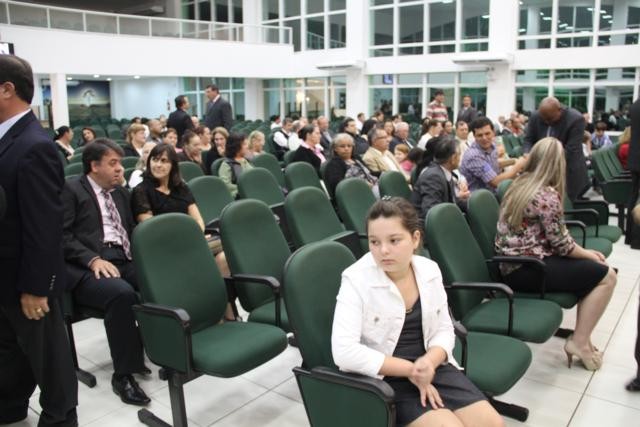The image is a detailed digital photograph capturing a large hall filled with dark olive green chairs, arranged in row after row. Among the seated audience, some individuals are seen standing, while others appear to be walking. At the forefront, centrally positioned, is a teenager wearing a striking red dress paired with a white jacket. She sits in one of the green chairs and looks off to the side thoughtfully. Toward the back of the hall, glass walls and doors frame the space, adding a backdrop of light and transparency. In the top left corner, a balcony-like structure is discernible. To the left of the image, a man dressed formally in a black jacket, white shirt, and black pants stands, contributing to an overall sense of formality. The attendees collectively wear a range of colors, reinforcing the notion of a formal gathering or event possibly related to a waiting area or ceremony.